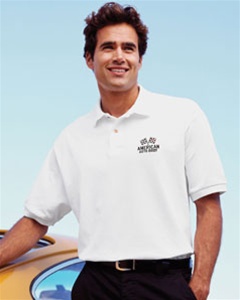In this professional or model photo, there is a tall Caucasian man with thick, bushy, slightly overgrown curly brunette hair and prominent eyebrows. He is dressed in a white polo shirt featuring a small logo of two overlapping checkered flags and the word "American." He pairs the polo with black slacks and a black leather belt with a silver rectangular design. The man stands leaning against a sporty yellow car, which is only partially visible, showing its low height and possibly the roof, windows, or hood and some lights. The man is facing and looking towards the right, with the photo's styling reminiscent of the late 90s or early 2000s.